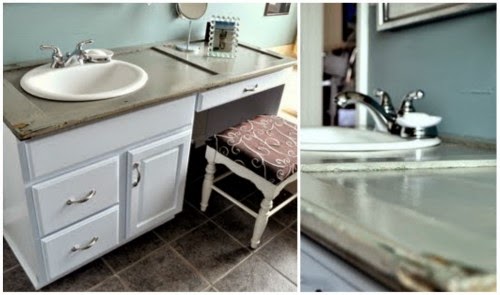### Detailed Caption

The image set includes two photos capturing different angles of the same bathroom vanity setup. The photo on the left presents a full view of the bathroom vanity, emphasizing its modern yet rustic design. The vanity is constructed with a white structure that includes two drawers and one cabinet. The surface appears to be made from an old door, characterized by its unique grayish-brown tone. A pristine white sink is seamlessly integrated into the countertop. To the left of the vanity, a maroon or burgundy cushioned stool is positioned, matching the overall decor. A long white drawer is placed in front of the stool for additional storage. On the countertop, beside the stool, lies a framed photo featuring a couple standing on the beach, adding a personal touch. A small makeup mirror is also situated on the counter, providing functionality.

The photo on the right offers a perspective from the point of view of someone sitting on the maroon cushioned stool, facing the vanity. This angle zooms into the centerpiece of the vanity – the white sink and its coordinating chrome faucet, showcasing the blend of utility and style in the bathroom's design.